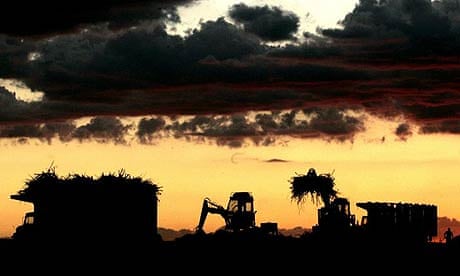The photo captures an evocative twilight scene set in an expansive field, during what appears to be evening as the sun sets. The sky is painted with hues of yellow, orange, red, and purple, juxtaposed against dark, looming storm clouds overhead. Below this striking sky, the landscape is teeming with activity: four work vehicles, including two trucks laden with hay and two bobcats lifting and depositing hay into the truck beds. One truck on the left is noticeably full of hay, creating an interesting contrast with the nearly silhouetted dark forms of the trucks and hay. Adding to the depth of the scene is a shadowy figure of a man standing behind a truck in the far right corner, contributing to the narrative of early rising farmers hard at work. The entire scene is both calming and emotionally moving, balanced perfectly between the vivid colors of the twilight sky and the dark, shadowed earth below.